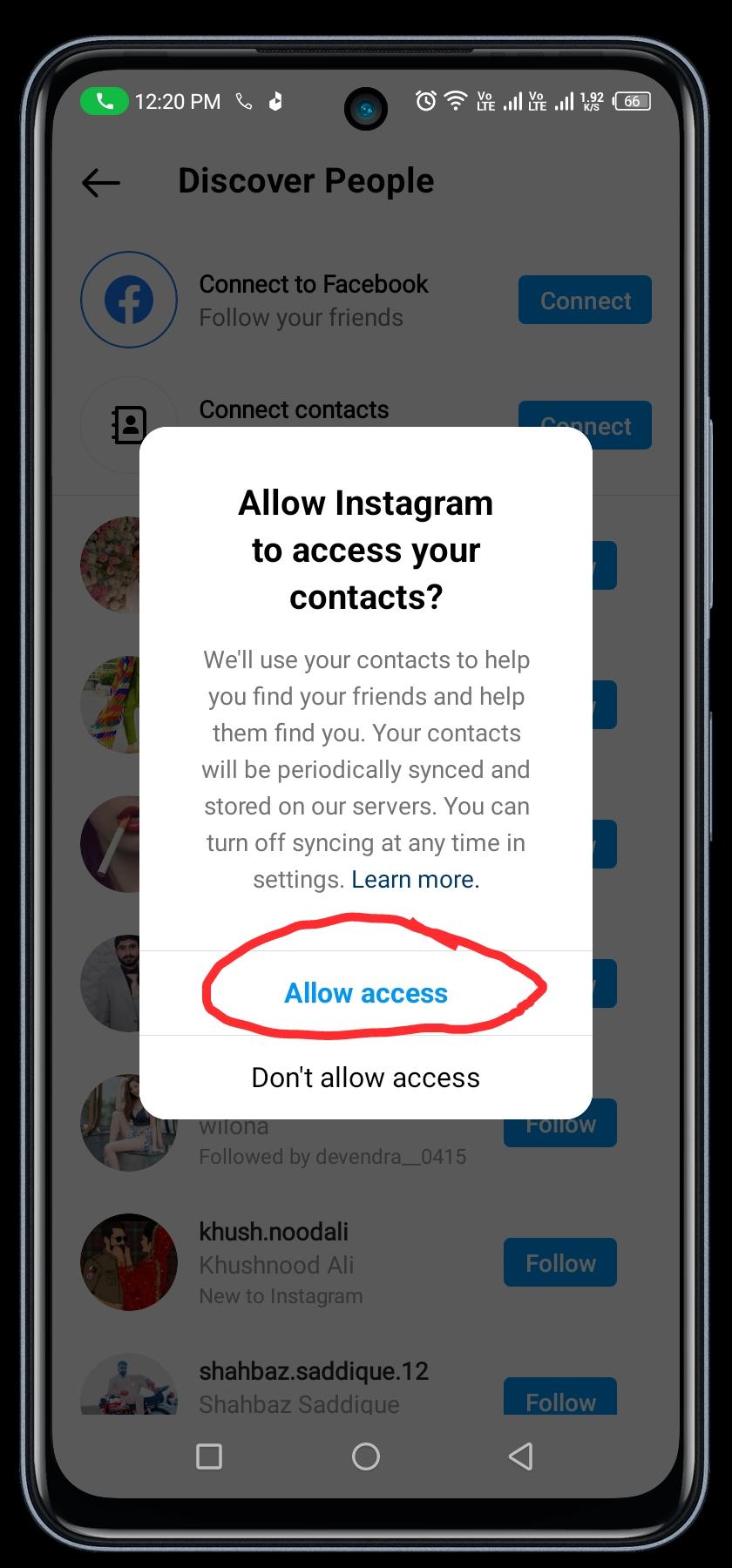The image portrays an illustration of a cell phone set against a black background. The phone itself has a sleek, black, shiny bevel. On its right side, there is a prominent large button, with a smaller button situated directly below it.

The phone screen displays a white webpage populated with various profile pictures, names, and blue buttons with white text. However, a notable feature of the screen is a white, vertically rectangular pop-up with rounded corners, obscuring much of the webpage.

At the top center of the pop-up, in bold black text, it reads, "Allow Instagram to access your contacts." Below this, there is a paragraph of medium gray text in a small font size: "We'll use your contacts to help you find your friends and help them find you. Your contacts will be periodically synced and stored on our servers. You can turn off syncing at any time in settings," followed by a blue "Learn more" link.

A thin light gray line runs horizontally beneath the paragraph. Below this line, blue text stating "Allow access" is awkwardly circled in a red oval. Another thin gray line appears just below this.

At the bottom of the pop-up, black text reads, "Don't allow access."

In the background of the webpage, at the bottom of the screen, are three white icons. On the left is a square outline with rounded corners, in the center is a circle outline, and on the right is a triangle outline with its tips oriented such that one points left, one up, and one down.